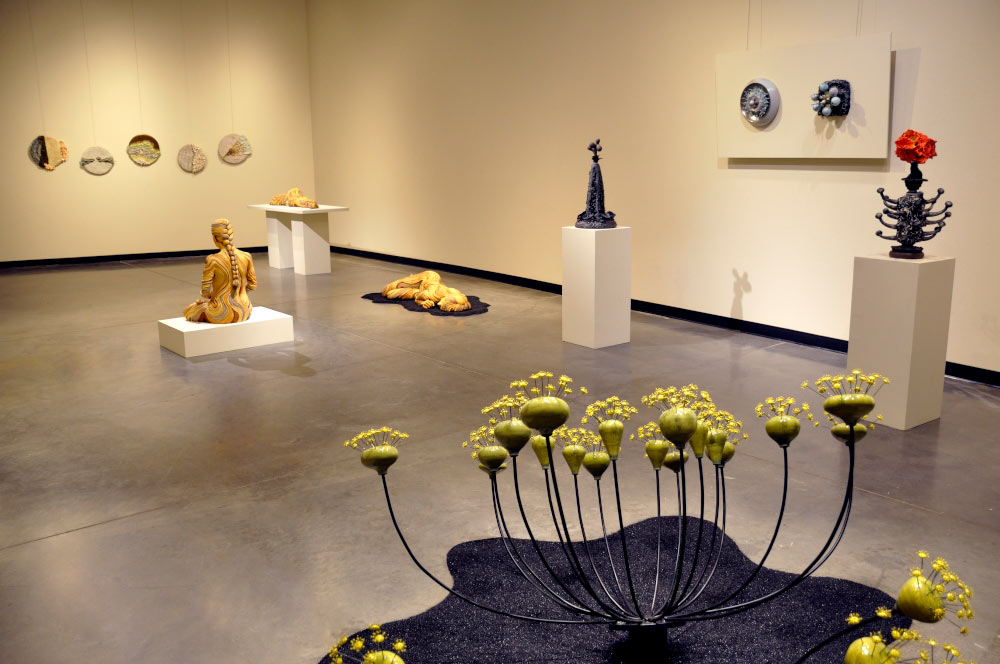The image depicts an art gallery with walls painted a beautiful ecru, creamish white. Along the far left wall, five circular disks - likely ceramic art - are suspended by cords, each hanging individually and displaying various types of artistic designs. Adjacent to these disks, a pedestal stands showcasing unique structures resembling coral formations.

Toward the bottom left, there is a striking female statue, sitting naked on a white rectangular podium, her back to the viewers. The statue features horizontal waves of colors and sports a long, gold ponytail. To the far right of these displays, a less distinguishable abstract structure lies on the floor, vaguely resembling hands or appendages, surrounded by a black, curved rug.

Moving further to the right, various pedestals display unique, multi-arm art objects and abstract black sculptures. One prominent sculpture is a black structure with blooming metal sections adorned with yellow, flower-like elements on top, positioned atop a black form-fitting rug. In the background, a highly detailed figure with a braid, formed with swirls of different colors, faces the wall with the circular displays. This dynamic and diverse collection of artworks, from intricate ceramics to vibrant sculptures, creates a rich, modern art experience within the gallery space.